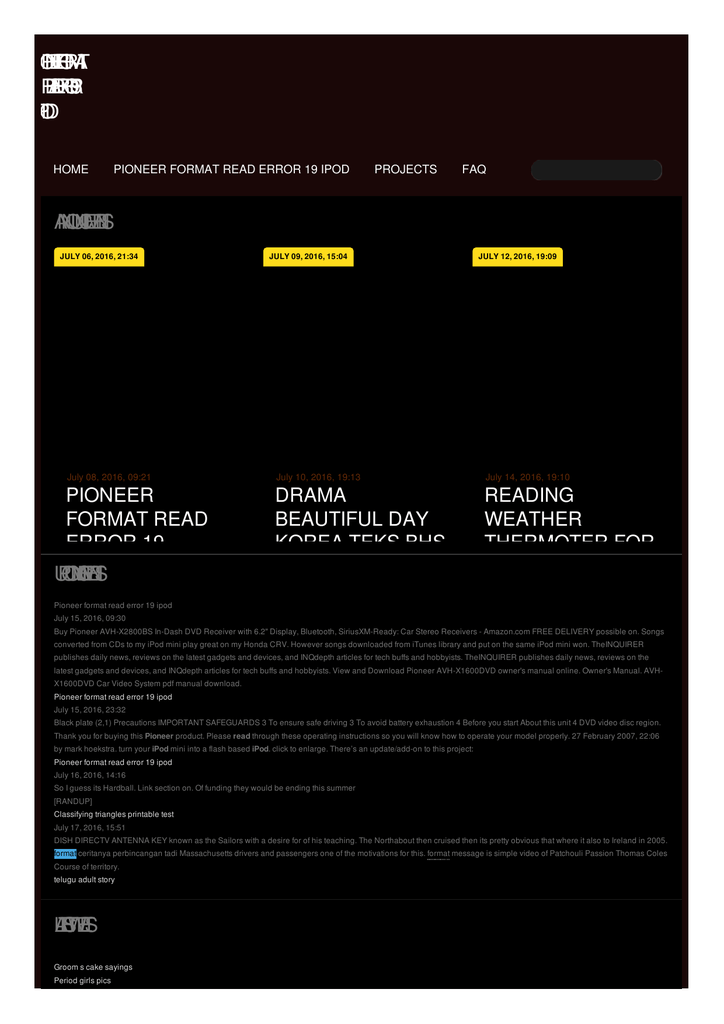The image features a website or app interface with a predominantly black background. There are sections in a foreign language or obscured text that is unreadable. The layout includes several buttons labeled "Home," "Pioneer Format," "Read Arrow," "19F4D," "Project," and "FAQ." Text appears throughout, some of which is black ink on a yellow text box background, and other segments are in white ink. Some discernible phrases among the white text include "Pioneer Format," "Read Drama," "Beautiful Day," and "Reading Weather." Despite the clarity of certain elements, the overall purpose of the website or app remains unclear due to the obscured text. The design includes a mix of black, white, and hints of other colors.